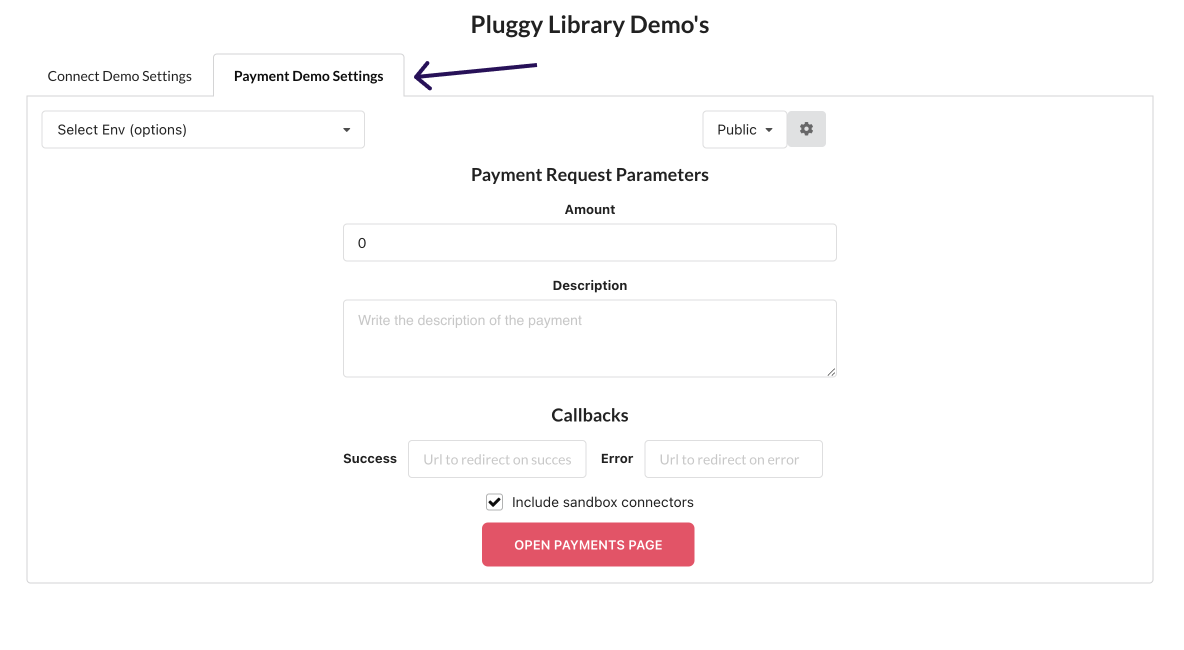Caption: 

In this screenshot of a settings interface, there are two primary options available for interaction: "Connect Demo Settings" and "Payment Demo Settings." The user has clicked on "Payment Demo Settings," which has expanded to display more details. An edited arrow points towards "Payment Demo Settings" with the label "Plug East Library Demos."

The expanded "Payment Demo Settings" provides a detailed configuration. It instructs the user to select their EMV (Europay, Mastercard, and Visa) options via a submenu located in the top left-hand corner. Additionally, towards the middle-right section, the user can find "Public Settings," which offers options to make the information public or private.

Further details outline "Payment Request Parameters," where the user can specify the amount, a description of the payment's purpose, and settings for callbacks. This includes URLs for redirection upon successful payments or errors. The settings also mention the inclusion of sandbox connectors.

At the bottom of the page, a pink-red button labeled "Open Up Payments Page" invites the user to navigate to a dedicated page for setting up payment processes and related configurations.